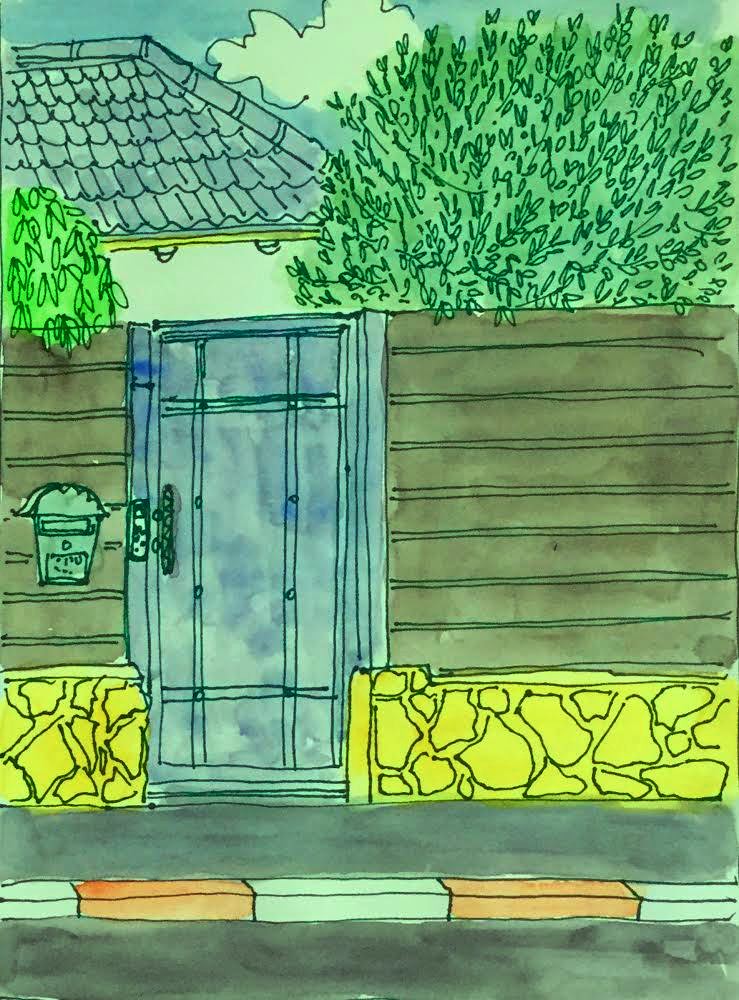The illustration depicts the facade of a house with a distinctive wooden fence in the foreground. The fence is composed of horizontal brown planks, resembling a solid wall rather than a traditional picket fence. Central to the fence is a blue door, secured with visible locks, and to its left hangs a small box, presumably a mailbox. The base of the fence is adorned with yellow stone sections, providing a contrast to the wood. In front of the fence, a gray sidewalk is bordered by red and white blocks, demarcating it from the street. Above the fence, treetops peek over, and a blue-roofed, white house is partially visible. The scene is completed with a bright blue sky and a single white cloud, adding to the serene suburban setting.